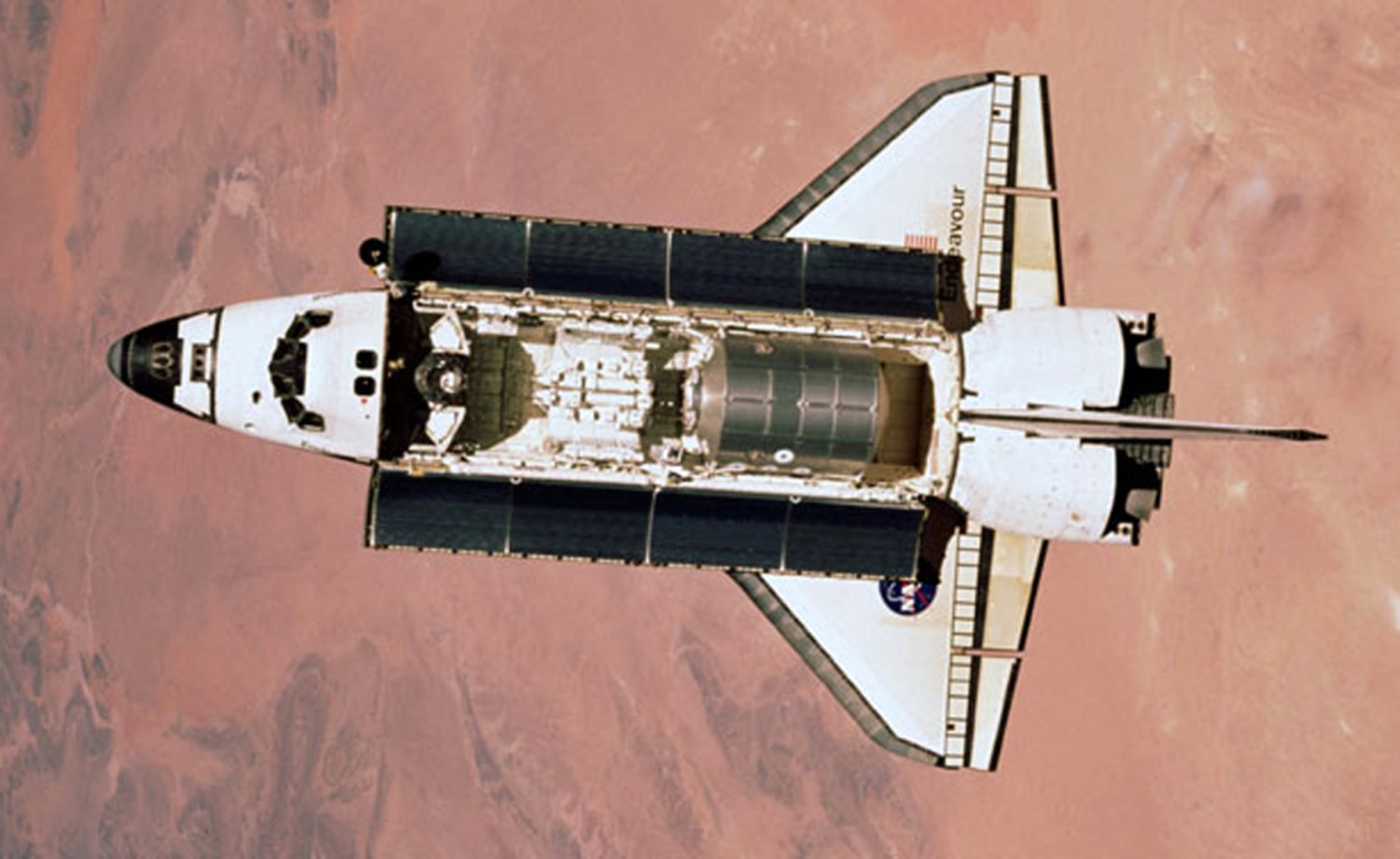This image showcases the space shuttle Endeavour from a top-down perspective as it orbits above a planetary surface. The shuttle, predominantly white with black trim, has two black panels and an open compartment that reveals its internal components, including a cylindrical metal object. The NASA logo and a partially visible American flag adorn the shuttle, with the letters "EA-V-O-U-R" confirming its identity as Endeavour. The background depicts a reddish, desert-like terrain, possibly hinting at the surface of Mars or a similarly arid planet, with swirling hues of reddish-brown and some purple. The photo, rectangular and seemingly taken from a close overhead angle, offers a detailed, almost hovering view of the shuttle against the striking planetary expanse below.